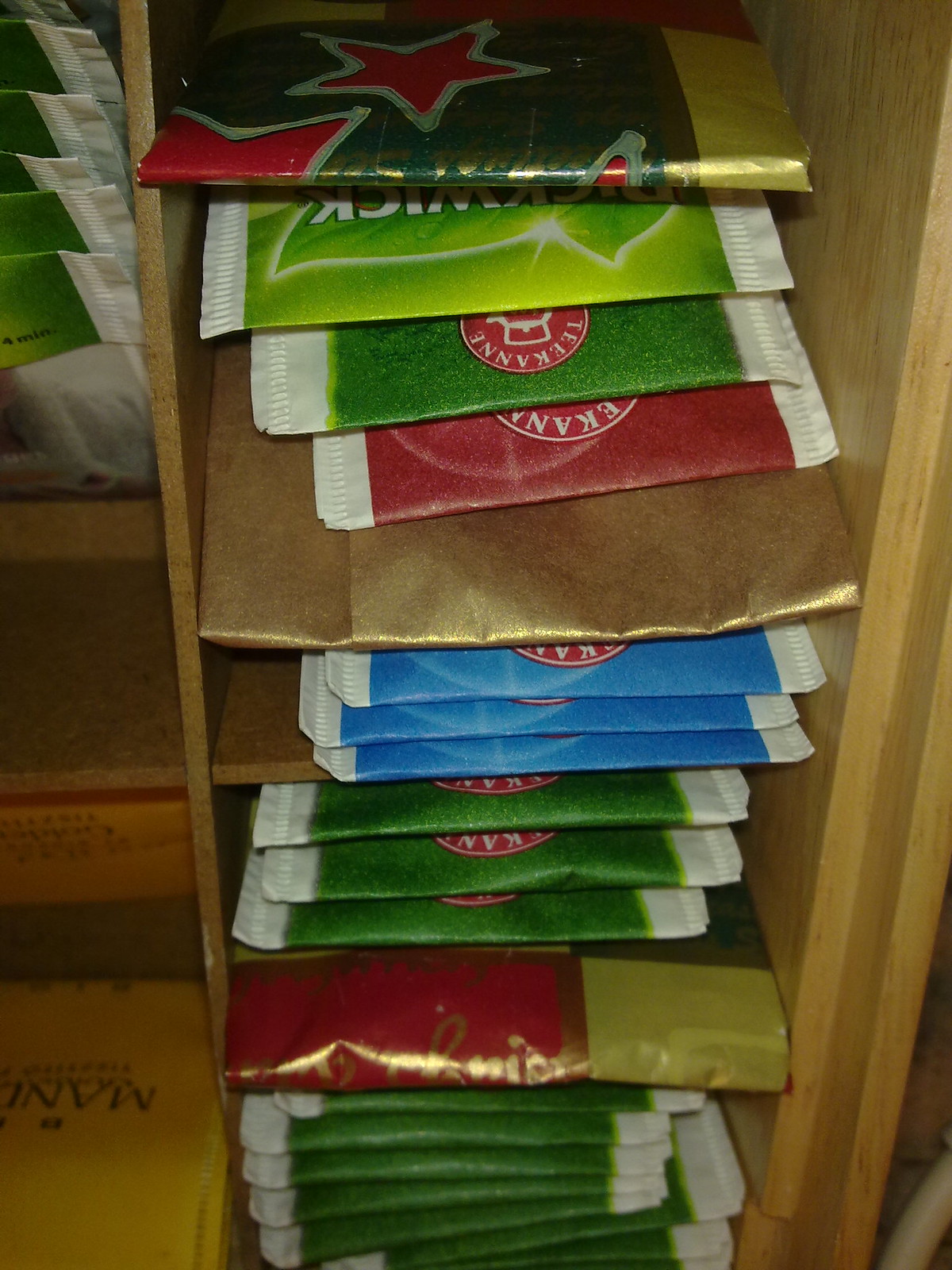This close-up, portrait-style photograph captures a wooden cabinet shelf stacked with an array of individually packaged teabags. The shelf is organized in single layers, each holding teabags of various colors, predominantly green, blue, and red. The teabags are of different brands and packaging styles, with many bearing the brand name "TEEKANNE." With roughly 20 varieties visible, each teabag is square-shaped, contributing to the uniform yet colorful display. The teabags are meticulously arranged in rows across multiple levels. The image highlights both the diversity and the systematic organization of the teabags on the shelf.